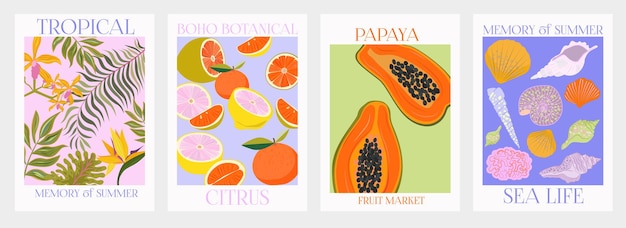This is a photograph of a grid displaying four equally spaced, flat-design artwork illustrations, each with vivid colors and thematic elements. The first image, titled "Tropical Memory of Summer," features a pink background adorned with various tropical plants, including palm branches, ferns, and bright yellow lilies. The second illustration, "Boho Botanical," presents a blue background with the word "Citrus" at the bottom, showcasing an assortment of citrus fruits such as lemons, limes, grapefruits, and oranges, both sliced and whole, along with green leaves. The third poster, labeled "Papaya Fruit Market," depicts a green background with a halved papaya, vividly orange with black seeds. The final illustration, "Memory of Summer Sea Life," set against a purple background, includes a variety of colorful seashells in different shapes and sizes.